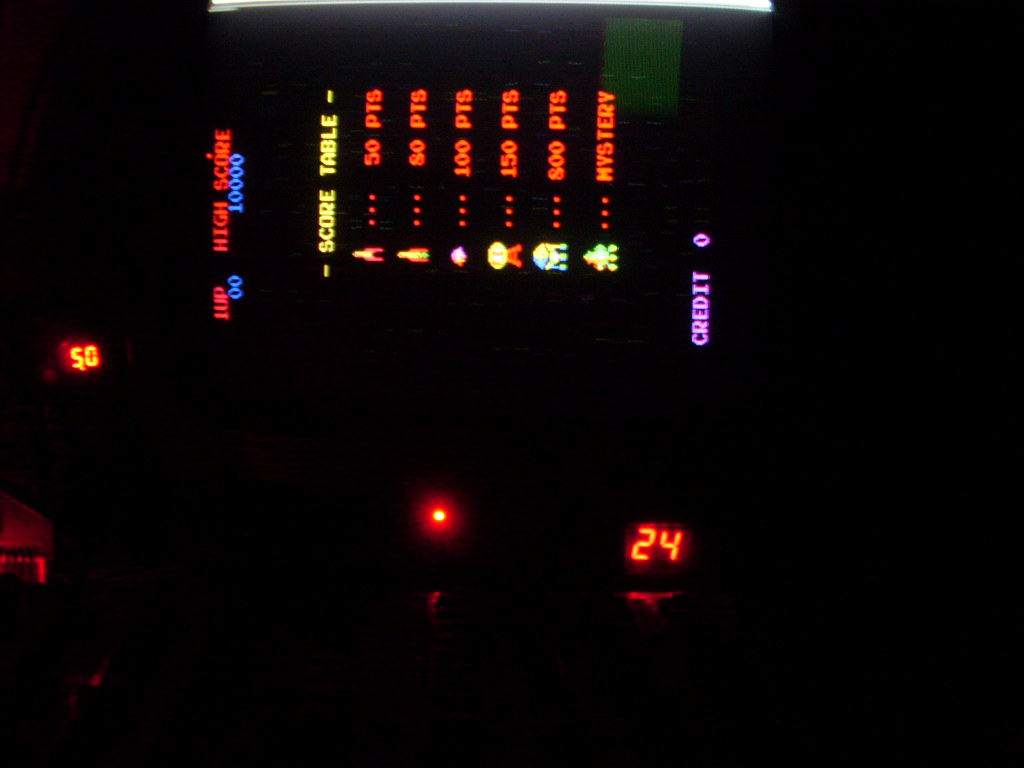The image appears to depict a scene reminiscent of the classic arcade game "Space Invaders." However, the television screen displaying the game is tilted awkwardly on its left side, making the view unconventional. The left side of the image is shrouded in darkness, but an orange glow highlights several important details.

Below the noticeably dark television screen, the number "50" is visible in this orange-red hue. A subtle red dot suggests that the device is powered on. To the right of the screen, the number "24" glows in a similar red-orange light. 

I had to tilt my head to read the text properly, and it states "1UP HIGH SCORE" in red, indicating the player's current status. Next to this, it shows "LIVES: 0" and "SCORE: 10,000." Further down, the score table is displayed, listing different objects and the corresponding points they offer when shot.

At the bottom of the screen, the word "CREDIT: 0" is written in a soft lavender color, indicating that no credits are remaining to play the game.

The image, though dark and tilted, captures the nostalgic essence of a "Space Invaders" gaming session.